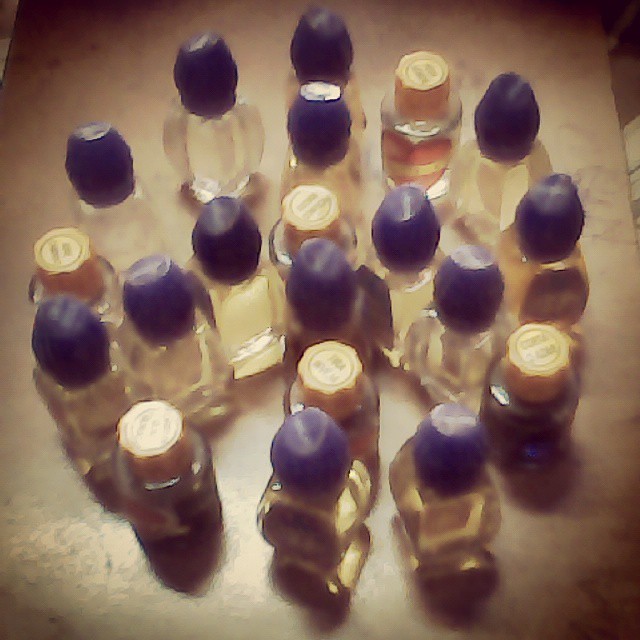The image is a blurry and out-of-focus shot of approximately 20 small bottles, likely perfume or fragrance bottles, clustered together on a tabletop that appears to be a yellowish beige or gold color. The tabletop is illuminated in the center, casting the outer edges into shadow. The bottles, each around 3-4 inches in height with a volume of about 5 to 10 milliliters, contain a clear or light yellow liquid. They have a mix of lid colors, with most bottles sporting roundish blue or purple caps, while others have flatter, gold-colored caps. Some of the bottles feature heart designs on the fronts, although any text or writing on the lids remains illegible due to the image's low quality.